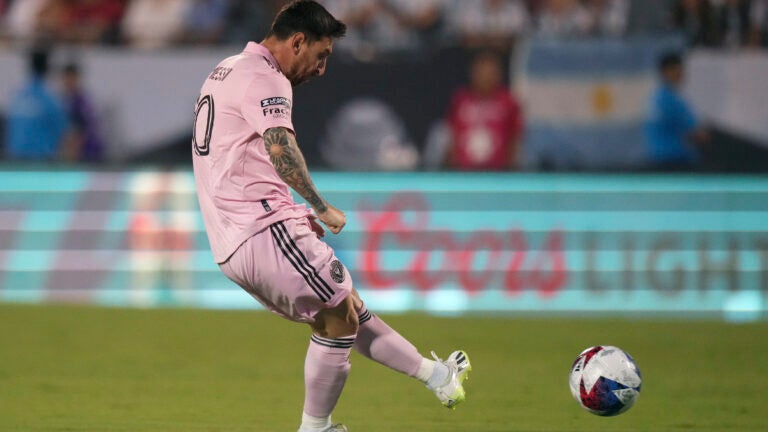In this dynamic image from a soccer event, Lionel Messi is captured in the midst of action on the pitch. Dressed in a pink jersey, white shorts featuring thin black stripes, white cleats adorned with neon green, and long white socks with shin guards underneath, Messi stands out prominently in the center of the frame. His short, dark hair and slight 5 o'clock shadow are clearly visible, as is the intricate tattoo extending up his left forearm to his elbow. With his left leg fully extended towards the ball—suggesting he has either just kicked it or is about to receive it—Messi intensely focuses on the round, white ball marked with sharp red and blue geometric shapes, hovering inches above the green field. The background, although blurry, shows a crowd in the stands, various observers, and advertisements for Coors Light along a blue barricade. Additionally, an Argentine flag is noticeable hanging from the front of the stands, adding a touch of national pride to the scene. Despite the blur, the vivid action and elements of the soccer event, with Messi at the forefront, are strikingly detailed.